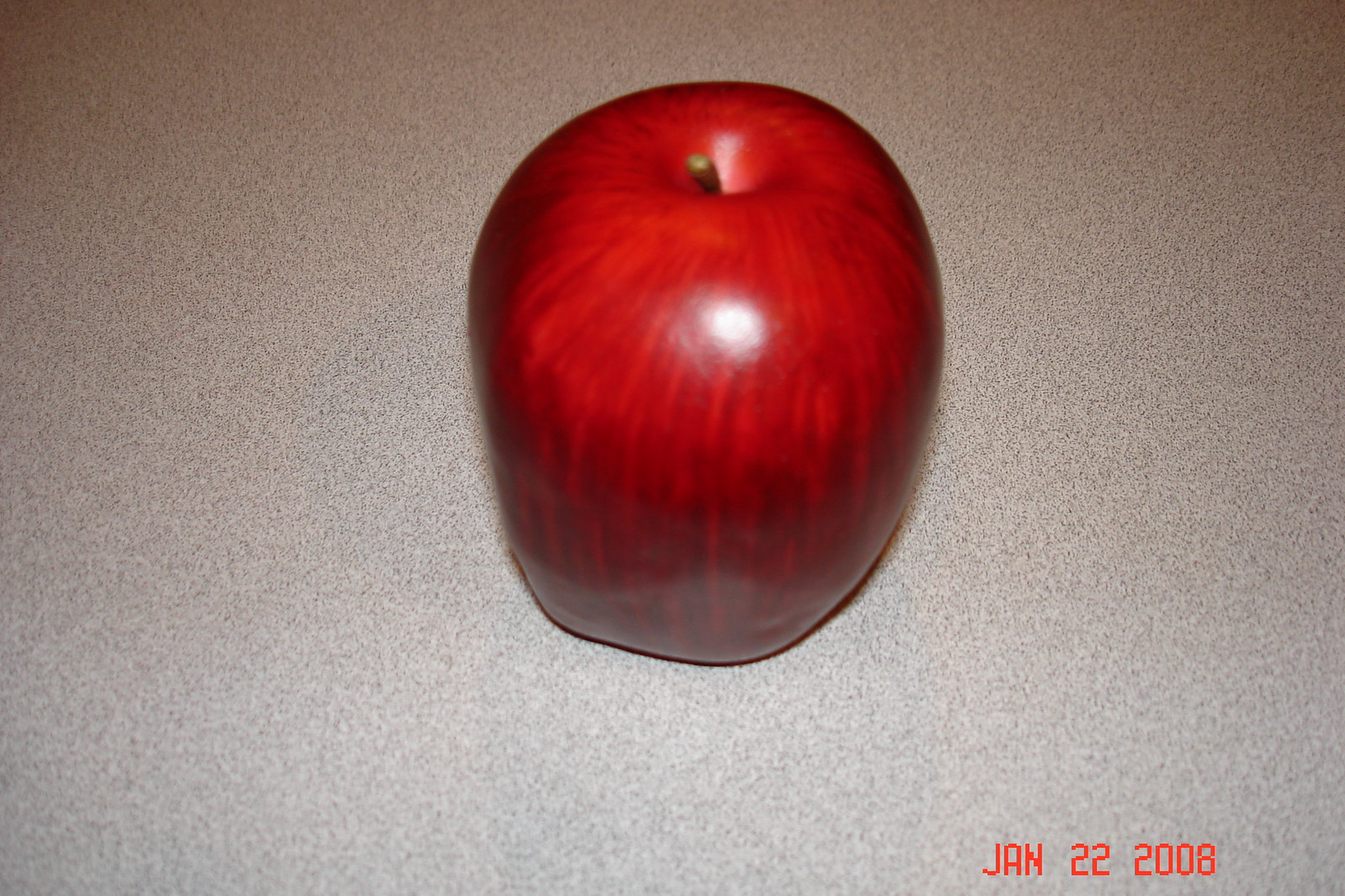A vivid photograph captures a single, untouched apple resting on a grainy, pinkish-brown tabletop speckled with black dots. The apple itself is a striking bright red, with a glossy surface reflecting the flash from the camera. The illumination from the front highlights the top of the apple, leaving it a lighter, vibrant red, while the bottom appears a darker, almost brownish-red with some black spots. A small stem protrudes from the top of the apple, nestled in a depression. The composition focuses solely on the apple against the distinctive tabletop, with no other objects or people present in the frame.